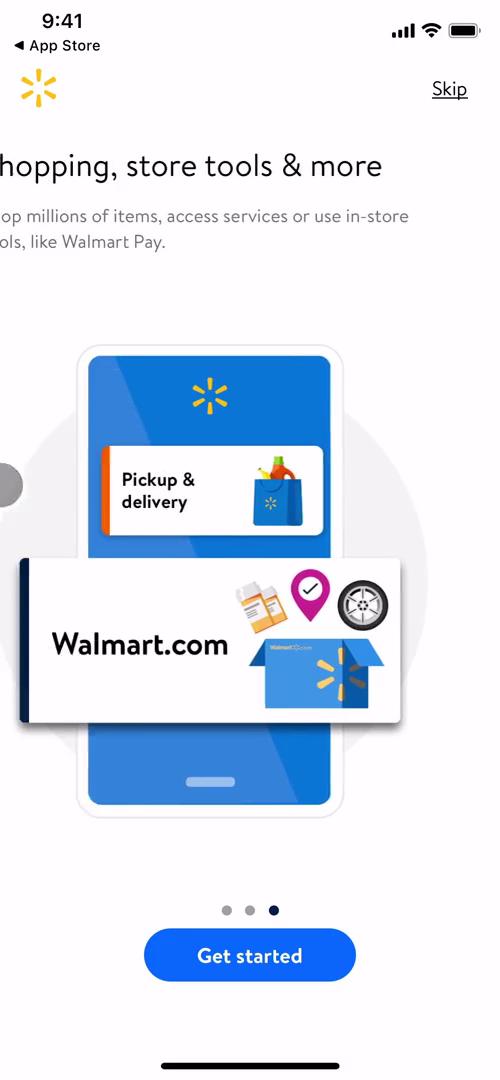The screenshot of a cell phone displays several key elements at the top of the screen. On the upper right-hand side, the Wi-Fi icon is fully lit, indicating a strong connection. Adjacent to it is the cell phone reception icon, also showing full bars, and the battery icon, which is completely charged. The current time is 9:41 AM, located on the upper left-hand side.

Below the status indicators, the screen shows the App Store interface with a back arrow to return to the previous screen. The Walmart logo, characterized by a sun symbol, is prominently featured to the left of a "Skip" button in the same row.

Just beneath these elements, a bold black font reads, "Shopping Store Tools and More." Below this, in smaller text, it states, "Millions of Items, Access Services, or Use in Store," followed by "OLS, like Walmart Pay."

At the bottom of the screenshot is an icon depicting a basic image of a cell phone. In front of this icon, there is a white box containing the text "Walmart.com." This comprehensive layout effectively combines key status indicators with a detailed view of the Walmart app's features and navigational tools.